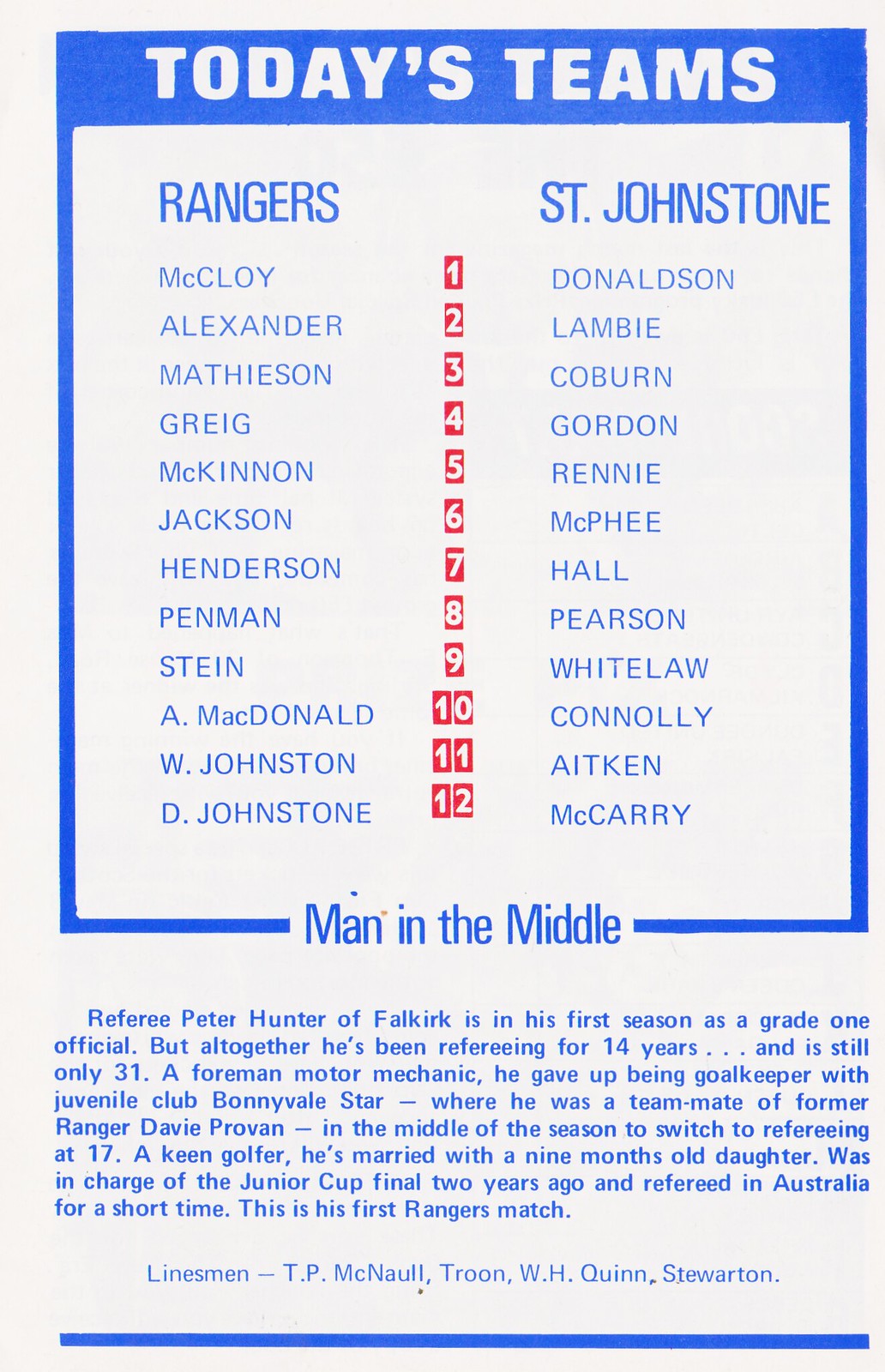This image showcases a sports program page with a predominantly white (slightly off-white) background and blue text. At the top, within a blue rectangle, white text declares "Today's Teams." Below this header, the content is arranged into two columns. The left column is titled "Rangers" and lists players by last names: McCloy, Alexander, Mathieson, Greg, McKinnon, Jackson, Henderson, Penman, Stein, A. McDonald, W. Johnston, D. Johnstone. The right column, titled "St. Johnstone," similarly lists the players: Donaldson, Lamb, B. Coburn, Gordon, Rennie, McPhee, Hall, Pearson, Whitelaw, Connolly, Aitken, McCary. Separating these columns are white numbers on a red background, numbered 1 to 12. Below the player listings, a section titled "Man in the Middle" provides a detailed paragraph about Peter Hunter from Falkirk, noting that despite it being his first season as a Grade 1 official, he has 14 years of refereeing experience and is still only 31 years old. At the bottom of the page, the linesmen are listed: T.P. McNeil from Troon and W.H. Quinn from Stewarton, with a decorative blue line finishing off the design.